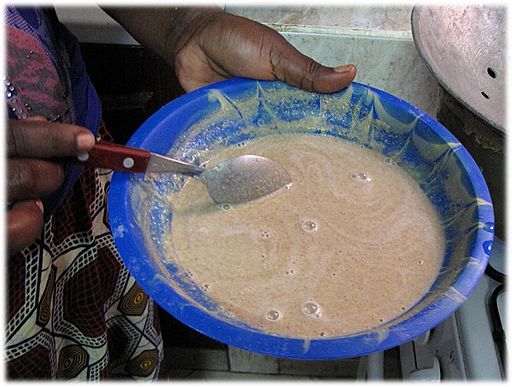In the image, a woman, possibly of African descent, is holding a dark purple-handled spoon with a silver spoon portion, while stirring a brown, bubbling liquid—likely a soup—contained in a blue bowl. Residue of the liquid marks the sides of the bowl. She appears to be wearing a skirt with a brown and white pattern. To her right, a grey metal bowl is visible. In front of the blue bowl, a white stove can be seen, along with white knobs positioned beneath the bowl and a white stove handle. The cooker surfaces align with the base of the bowl. To the left, there is a dirty white counter that slightly slopes down and becomes flat around the level where her wrists are positioned.